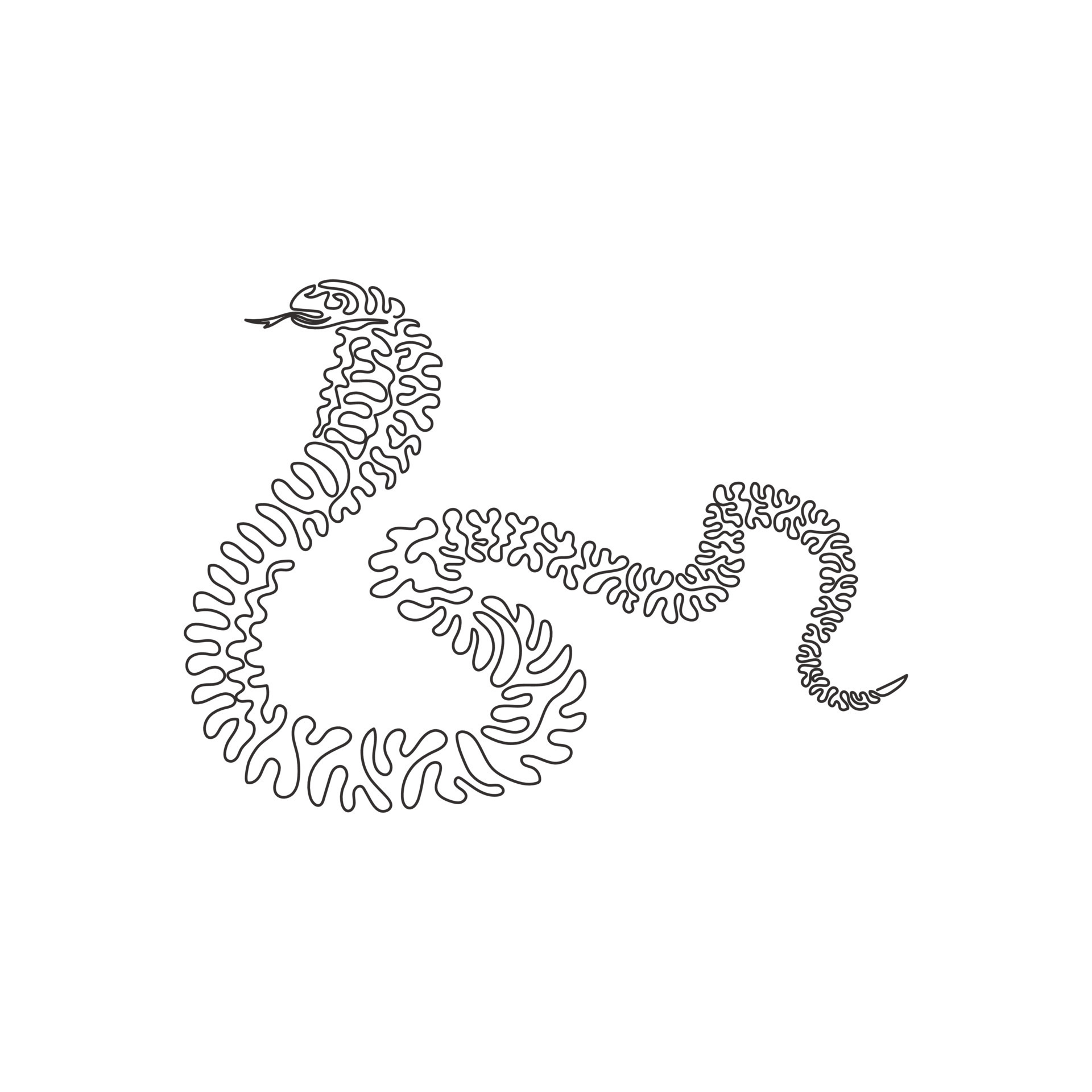This image is a detailed black and white abstract drawing of a snake on a white background. The snake's body, head at the top with a forked tongue sticking out and a pointed tail at the bottom, is composed of numerous swirling, swooping squiggly lines that coil in a puzzle-like fashion. The drawing is minimalistic, yet intricately designed to resemble a snake, likely a cobra, given the fan-like hood extending from its head. The snake's form is made from what appears to be a single continuous line, with occasional gaps suggesting eyes. The line curves downward, upward, left, right, creating multiple U-bends that simulate the winding, coiling motion typical of a snake. Despite the abstract nature, the cohesive linework clearly represents the reptilian form as it gracefully slithers across the white backdrop.